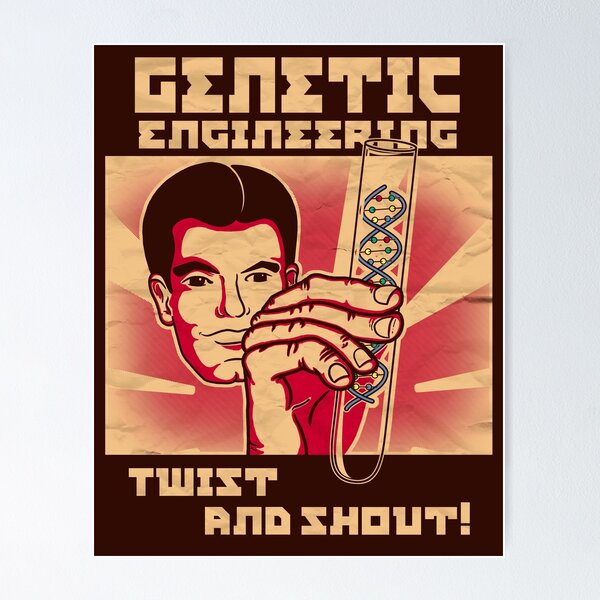This square-shaped, retro-style poster features a central drawing with thick brown borders at the top and bottom and thin dark brown borders on the sides. The top text reads "Genetic Engineering" in a light beige, almost cream color against a dark brown, somewhat red-tinted background, and has a vintage 1950s feel. Beneath this header is a striking depiction of a man's head, styled similarly to characters from "Mad Men," with slicked-back brown hair, dark brown eyes, dark eyebrows, and a subtle smirk. The man appears to be a genetic engineer, holding a test tube in his hand. Inside the test tube, there's a vividly drawn DNA strand intertwined with colors like blue, red, green, and yellow. The background of the central image features a light brown area with a red blotchy effect emanating from the center, reminiscent of sun rays. Below this image, in matching beige text on a brown background, the poster exclaims "Twist and Shout!" giving it a kitschy, nostalgic vibe. The entire composition, including its dimensions of approximately four inches by four inches, reinforces the whimsical and attention-grabbing nature of this artwork.